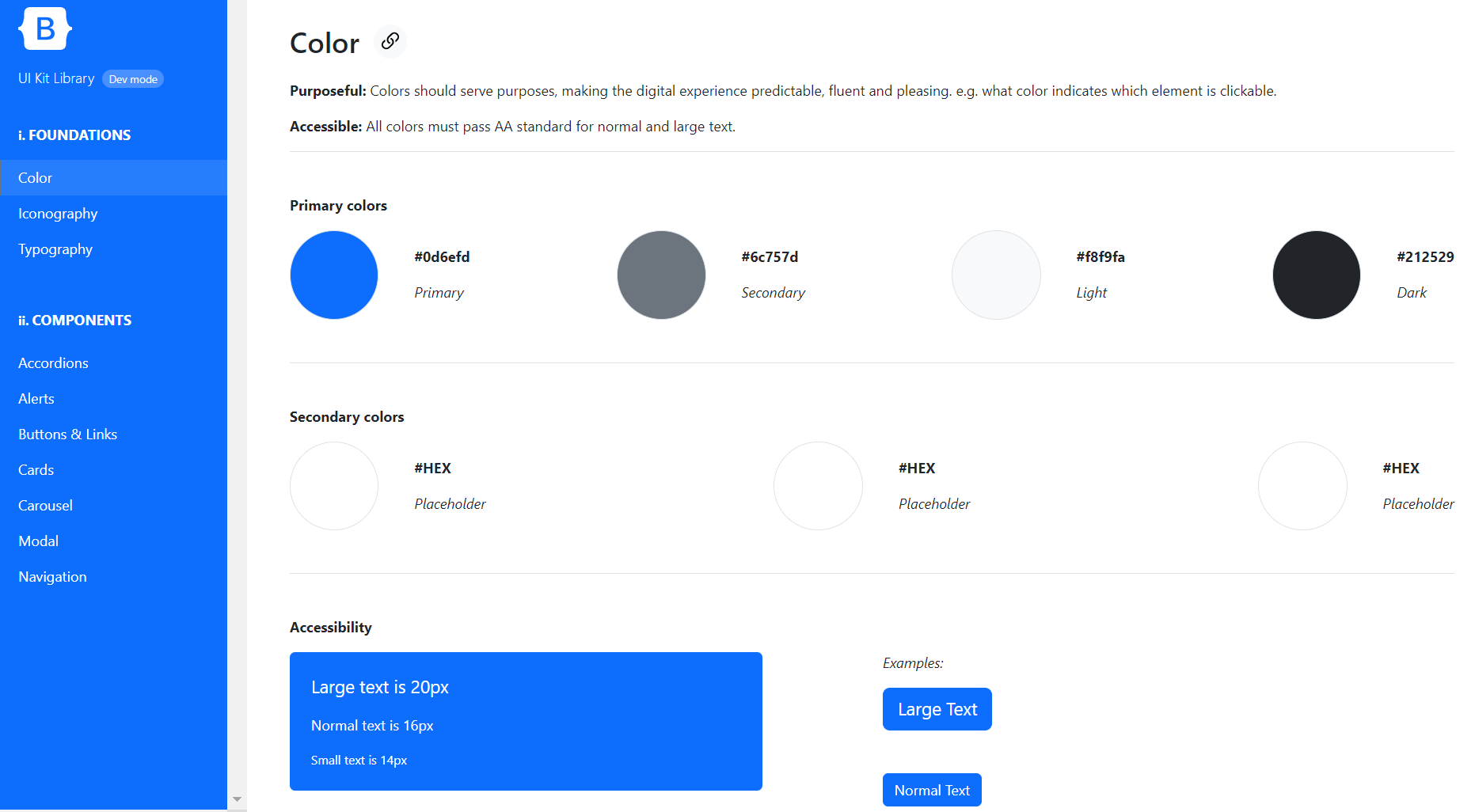The image depicts a digital interface, likely a website manager or UI kit library dashboard. On the upper left side, there is a vertical blue bar extending from the top to the bottom of the screen, featuring a white logo with a stylized blue "B." Below this logo, the title "UI Kit Library" is displayed. The navigation menu lists various sections including Foundations, which covers categories like "Color," "Iconography," and "Typography," and Components, which spans "Accordions," "Alerts," "Buttons and Links," "Cards," "Carousel," "Modal," and "Navigation."

On the right-hand side of the image, the background is primarily white. At the top, the word "Color" is prominently displayed, followed by descriptors "Purposeful and Accessible." Below this, two lists are presented: "Primary Colors" and "Secondary Colors." Additionally, there is a section dedicated to "Accessibility," which illustrates differences in text sizes with examples labeled "Large Text" and "Normal Text." The examples clearly demonstrate the visual distinctions and accessibility considerations between different text sizes.